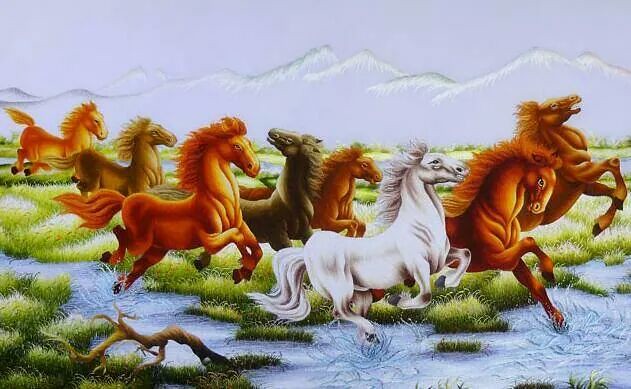This image depicts a beautifully detailed painting of an outdoor scene featuring eight wild horses galloping through a water-logged grassy field. The background showcases a light purplish-blue sky blending seamlessly with the white and green-tinted outlines of distant mountains. The ground plane is a marshy landscape interspersed with patches of green grass and blue puddles, alongside a notable brown tree branch on the left.

The horses are captured in various dynamic stances, all moving towards the right of the frame, their manes flowing freely. They come in a range of colors: the horse nearest the front is pure white, while the others are various shades of brown—from light to dark, including a dark brown horse and a reddish-brown one. Standing out amidst the group, the white horse adds a striking contrast to the darker tones of the others. This cohesive scene of natural beauty and fluid motion brings the wild and powerful essence of the galloping horses to life.